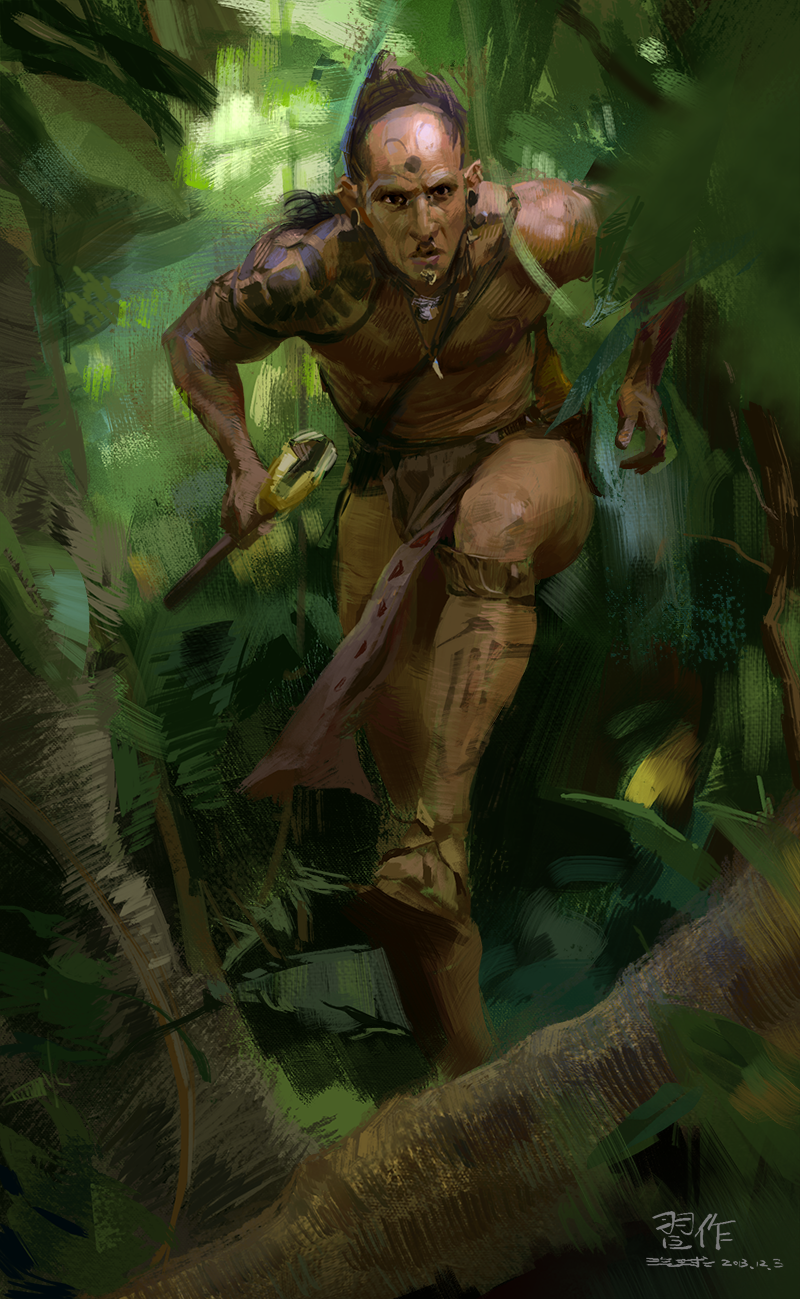The painting depicts an indigenous man dynamically running or trekking through a dense, vividly green jungle. The figure is captured mid-motion, with his right leg lifted, about to cross over a tree branch or log. His complexion is brown, and he has a distinctive hairstyle: the top half of his head is shaved while the rest of his hair is pulled back into a long ponytail. Notably, he has a prominent brown dot on his forehead and facial paint or tattoos in grey and black hues.

Adorned with traditional jewelry, the man sports large, round black disc earrings in both ears and a nose ring. His upper body is bare, save for a brown strap crossing his torso, likely connected to a shoulder bag. Intricate tattoos or paintings extend down his right shoulder and arm, further accentuating his indigenous heritage. Around his neck, he wears necklaces fashioned from what appear to be animal fangs or bones.

The man’s attire is minimal yet detailed, consisting of a brown loincloth with red triangular patterns that reaches his knees. His calves are decorated with markings or tattoos, and he wears brown braces just below his knees along with brown sandals to protect his feet. In his right hand, he holds a yellow-headed axe or mallet, emphasizing his readiness for survival or combat in the jungle.

Adding to the historical or cultural context of the artwork, the painting includes an inscription in the bottom right-hand corner. The script is not entirely legible but appears to be in characters that may represent an indigenous hieroglyph or an Asian language. The overall scene is richly detailed, with the lush greenery of the foliage surrounding the focused and powerful figure, suggesting a narrative of determination and connection to the natural world.